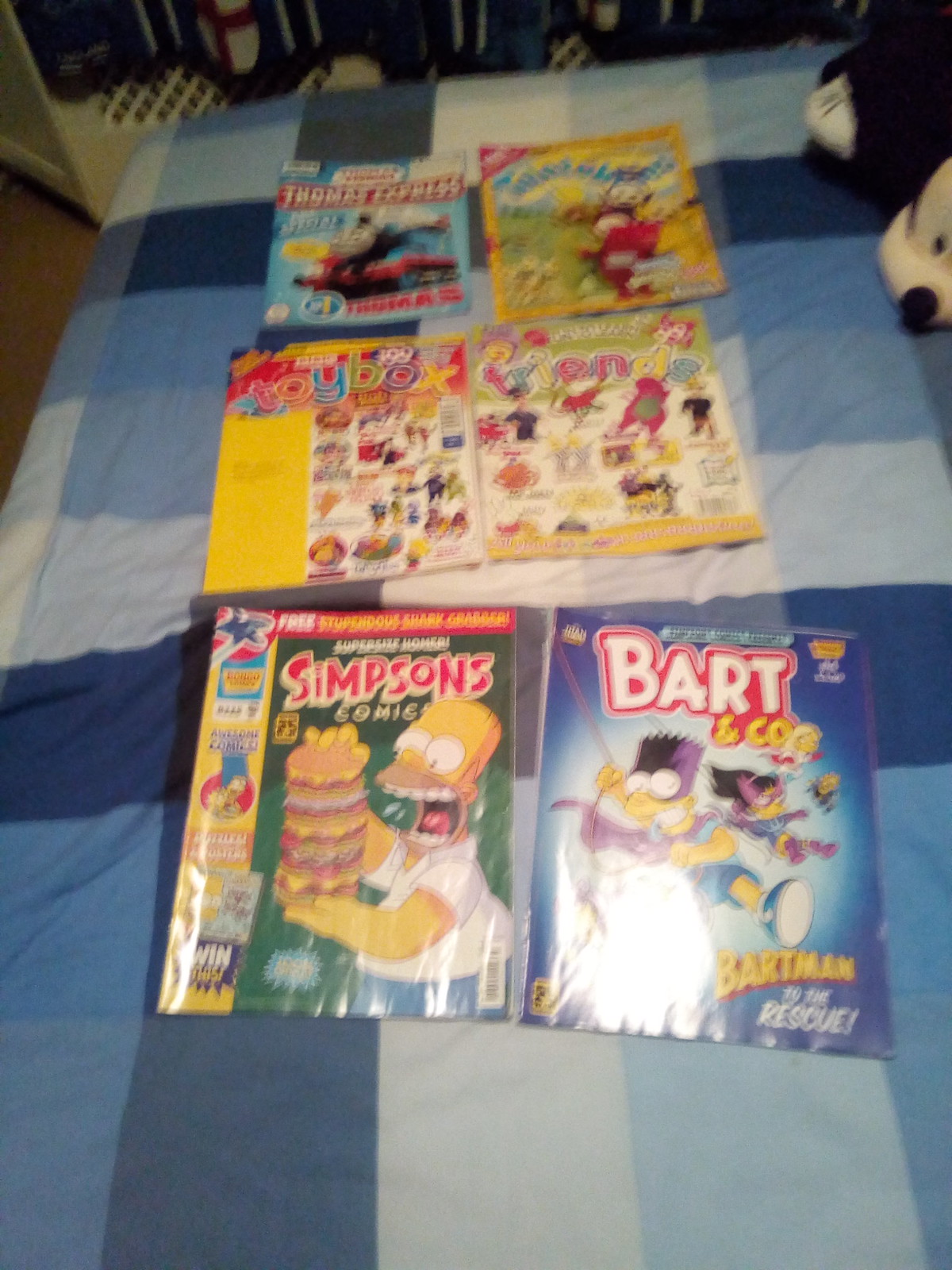This photograph captures a dimly lit child's bedroom featuring a bed covered with a plaid bedspread patterned in various shades of blue and white. Laid out meticulously on the wrinkled fabric of the bedspread are six children's comic books, arranged in two rows of three. At the bottom left, there's a "Simpsons Comics" issue depicting Homer Simpson devouring a towering burger that's taller than his head. Next to it is another Simpsons comic titled "Bart and Company," showing Bart Simpson in his Bartman superhero costume alongside a girl in a similar outfit. Moving upward, a yellow comic named "Teletubbies" and another titled "Toy Box" are placed side by side. At the top, a blue comic featuring Thomas the Tank Engine labeled "Thomas Express" sits next to a partially unclear comic that reads "Friends." To the right edge of the image, a Mickey Mouse plushie is partially cropped out, with only his face and part of his black clothing visible. The background reveals a simple white wall and a glimpse of a brown floor peeking out from the bed's left side.